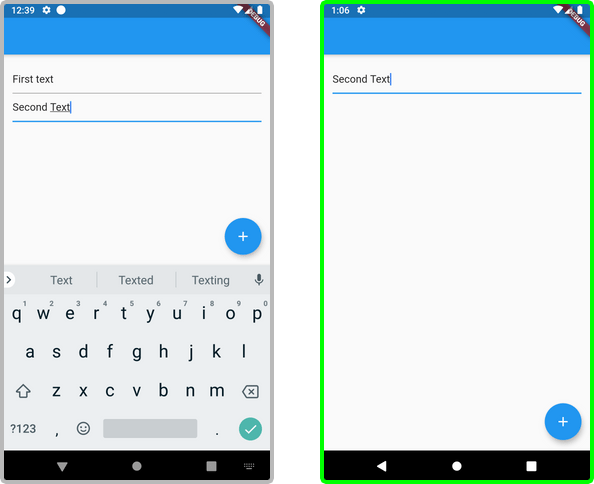The image consists of two mobile phone screenshots side by side. 

**Screenshot 1 (Left):**
- **Time Displayed:** 12:39, located in the top left corner.
- **Debug Indicator:** A small maroon banner diagonally placed in the top right corner of a solid blue header.
- **Main Screen Background Color:** Predominantly white.
- **Text Details:**
  - *First Line:* Reads "First text" in small black font.
  - *Line Divider:* A solid gray line beneath the first text.
  - *Second Line:* Reads "Second text," with "text" underlined and a cursor positioned after it, suggesting active typing.
- **Keyboard:** Visible at the bottom, featuring a standard phone keyboard layout with a lighter gray background.
- **Autocomplete Suggestions:** Displayed at the top of the keyboard, including "text," "texted," and "texting."
- **Navigation Bar:** A black strip at the bottom housing a triangle, a circle, and a square.

**Screenshot 2 (Right):**
- **Keyboard Absence:** The keyboard from the first screenshot is not present, making the entire screen appear white, except for the text.
- **Text Details:**
  - The text "First text" is missing.
  - A single line of text reads "Second text," with a green underline.
- **Green Border:** The entire screenshot is framed by a bright green border.

Both screenshots are nearly identical aside from the absence of the keyboard and the "First text" line in the second screenshot, along with the additional green elements in the latter.